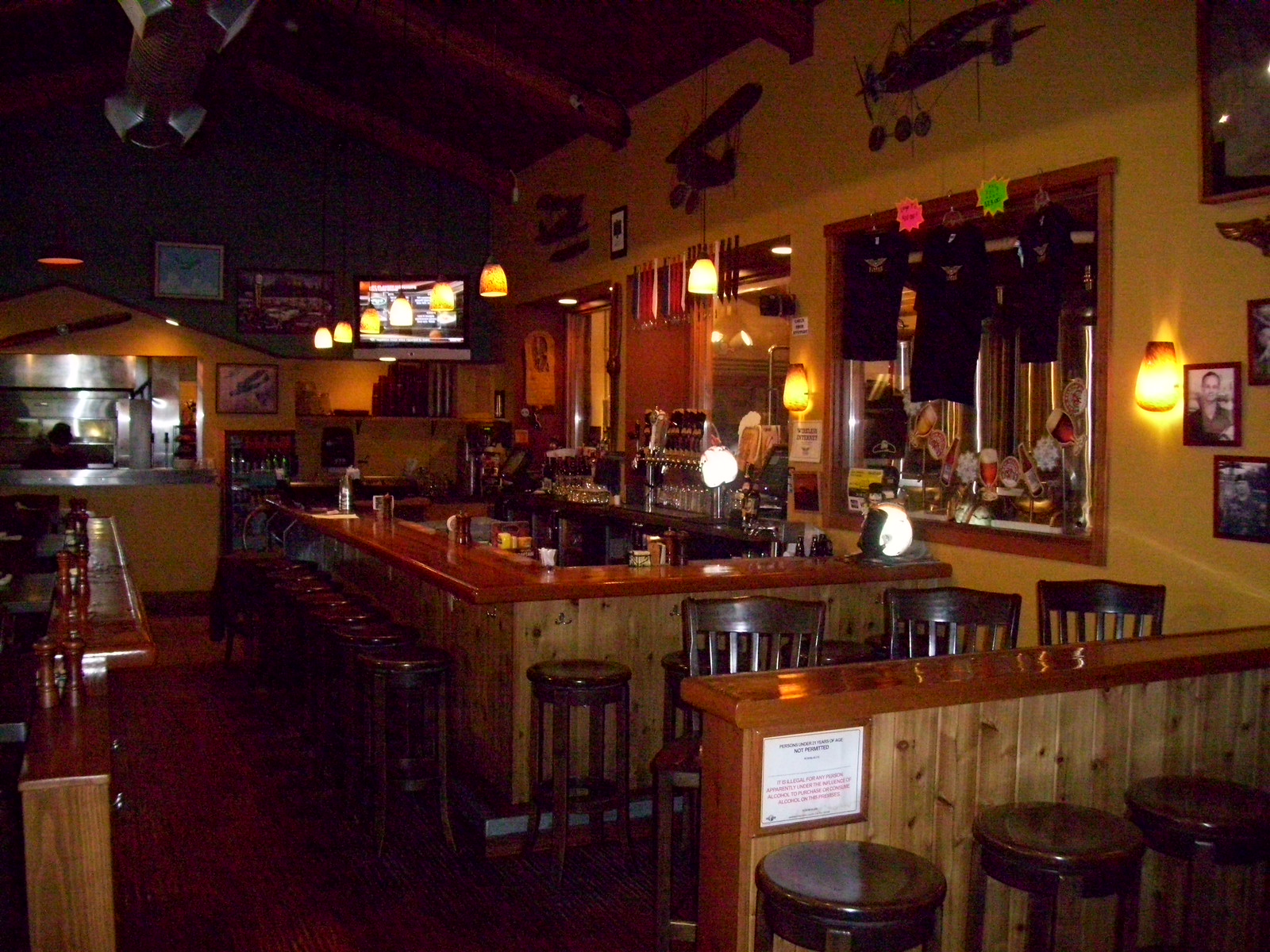The image depicts an inviting bar area, characterized by warm, earthy tones dominated by polished and stained brown wood. Central to the scene is a polished brown bar top, accompanied by a row of circular leather bar stools and additional brown bar chairs situated near a half wall with vertical wood paneling, offering extra seating. The atmosphere is dark and amber, enhanced by yellowish pendant lights and sconces on the walls. 

The bar itself boasts beer taps and an array of drinking glasses, indicative of its primary focus on beer rather than liquor. Condiments and napkin holders are neatly arranged on the bar surface. Mirrors line the back wall, reflecting the cozy ambience, while a TV hangs in the corner for entertainment. Framed illustrations of airplanes adorn the walls above and around the bar, suggesting a possible aviation theme, perhaps hinting at a location near an airport. Despite the lack of patrons in the image, the bar appears well-maintained and inviting, ready to welcome its next guests.